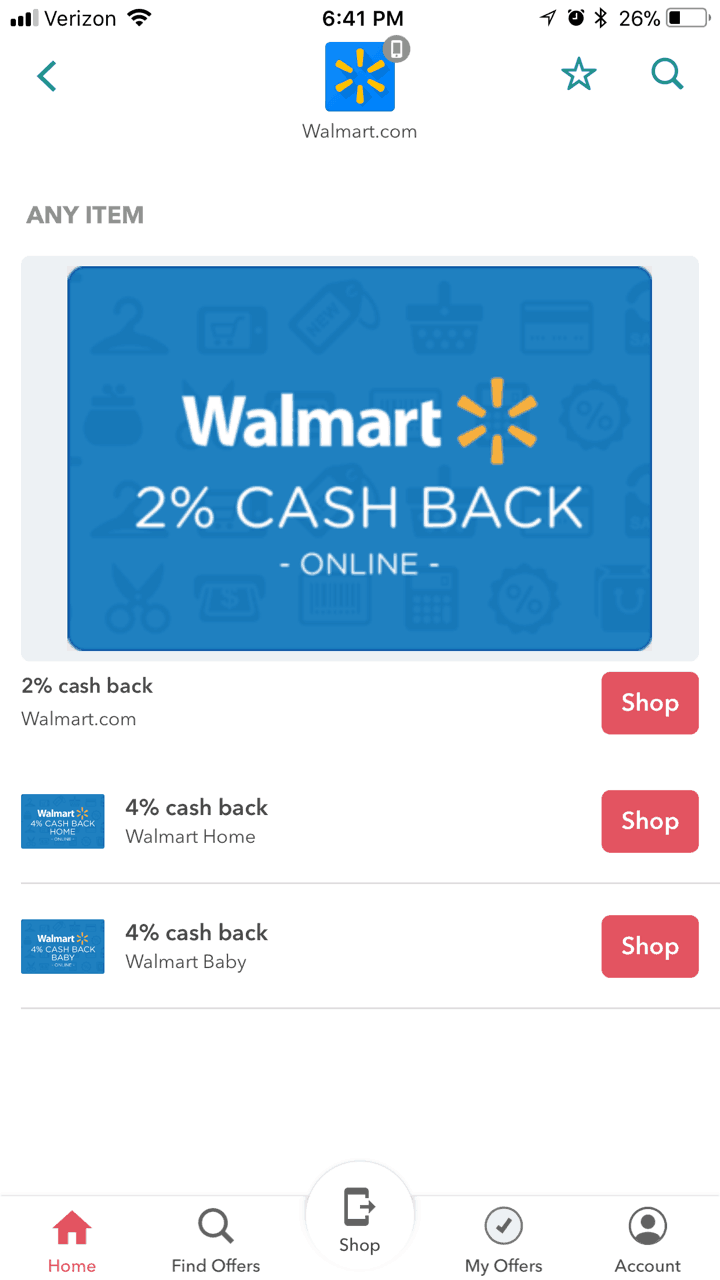The image depicts a cell phone screen displaying the Walmart.com mobile website. At the very top of the screen, the phone indicators reveal various status icons: the cellular signal strength shows four bars, with three of them highlighted in black, indicating Verizon as the service provider. A full Wi-Fi signal is present, and the time is indicated as 6:41 p.m. On the right-hand side, additional icons display the clock, Bluetooth status, and a battery level at 26 percent.

Centrally, a small square box features a yellow emblem resembling a sun, with the text "walmart.com" prominently displayed. In the left-hand corner, the phrase "ANY ITEM" is written in gray, all in capital letters. Below, a blue rectangular image represents a Walmart credit card marked with "Walmart" in white text and accompanied by the sun emblem. The words "2% cashback online" are situated beneath the "Walmart" logo.

Further descriptive text in gray reads "2% cashback walmart.com," situated beneath the credit card image. On the right-hand side, three small, vertically stacked red squares, each with the word "SHOP" written in white, are visible. On the left-hand side, another set of two blue rectangular icons, positioned side by side, represents additional categories. The first icon denotes "4% cashback walmart home," and the second specifies "4% cashback walmart baby."